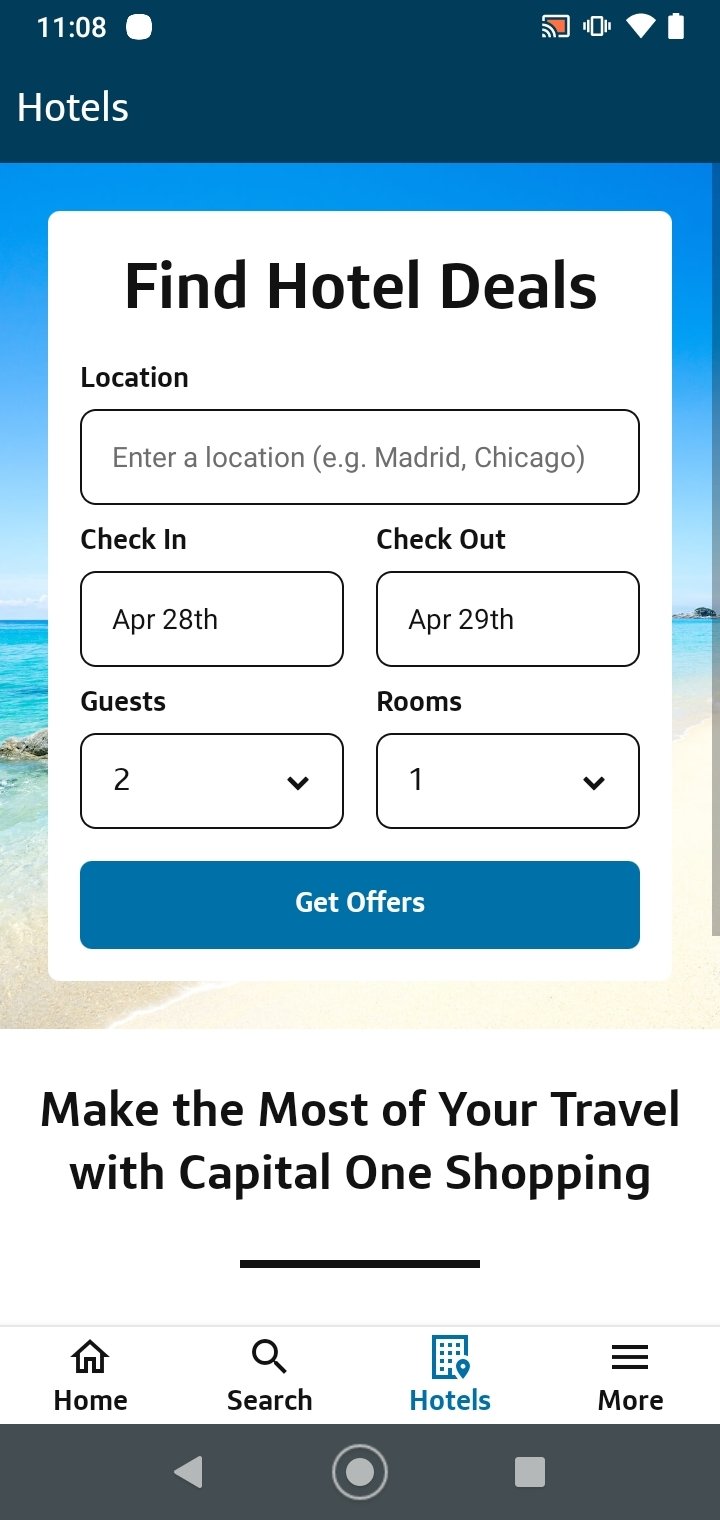The image captures a screenshot of a hotel booking interface from a mobile phone. At the top, there is a header titled "Find Hotel Deals." Directly below this header, a location input box is present where users can type in their desired destination. Following this, there are input fields labeled "Check-In" and "Check-Out," with the dates set to April 28th to April 29th by default, but users are able to adjust these dates according to their plans.

Next, the interface features a section for "Guests," which is currently set to two people, and another for "Rooms," which defaults to one room. Both sections include drop-down menus allowing users to modify the numbers according to their needs.

Towards the middle to the bottom area of the screen, a promotional message reads, "Make the most of your travel with Capital One Shopping." Below this promotional content, a horizontal grayish-black line divides the screen, beneath which four clickable icons are displayed: "Home," "Search," "Hotels," and "More."

At the very bottom of the image, a black rectangle contains three navigation icons: a triangle, a circle with an additional line around it, and a square. These icons likely serve as navigation buttons for the phone's interface.